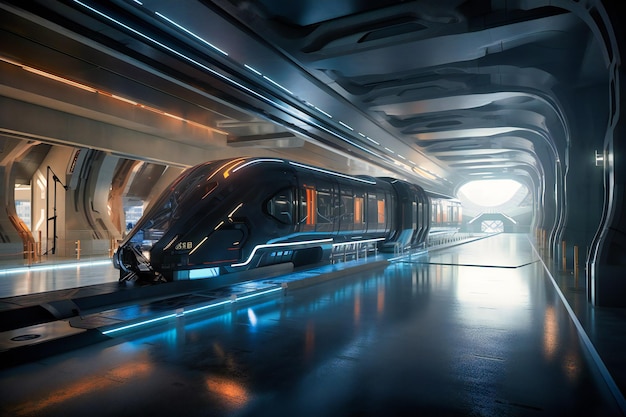The image portrays a sleek, futuristic train station illuminated by vibrant LED lights in blue and orange hues. The train, resembling a streamlined bullet train, appears to be levitating above its magnetic track. It features a dark, metallic blue exterior with reflective surfaces that catch the lights around it. The train is short, consisting of two main cars—one for the conductor and one for passengers—accented with vertical orange-lit windows. The station itself has a modern and sterile design, with smooth, metallic surfaces and curving, wavy walls and ceilings. There are no visible people, lending the space a clinical atmosphere. The ground is highly reflective, amplifying the glow of the station's lights. A bright opening at the end of the tunnel lets in natural sunlight, contrasting with the otherwise synthetic environment. The left side of the image shows a platform area for passengers, and multiple pillars adorned with intricate details line the right side. The overall impression is that of a highly advanced, sci-fi-inspired setting.